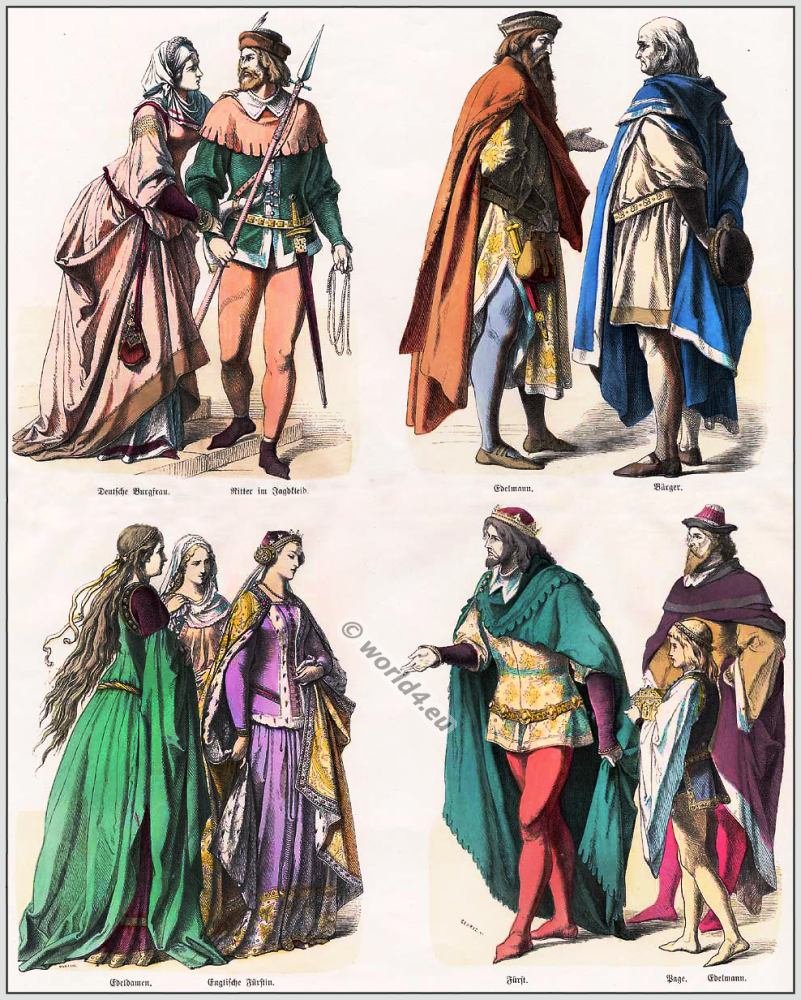This vertically rectangular, full-color artistic piece consists of four distinct images, each bordered by a very thin black line against a very light peach or off-white background. Each quadrant of the piece portrays individuals dressed in medieval attire. In the upper left corner, a woman in a long flowing pink dress and a kerchief stands beside a man in brown shoes, peach tights, a green shirt, and an orange hat, holding a spear. In the upper right corner, two men, one in a white tunic with a long blue robe and the other in a yellow dress with a red cape and blue tights, converse with each other. The lower left quadrant features three women adorned in Middle Ages garb — green, purple, and tan dresses. The lower right corner depicts two men, one wearing red tights, a golden shirt, and a green cloak, and another in a purple cloak, talking to three women in medieval dresses, while a young girl stands nearby. The artistic piece is marked with "C in a circle, world4.eu" in the bottom lower center.